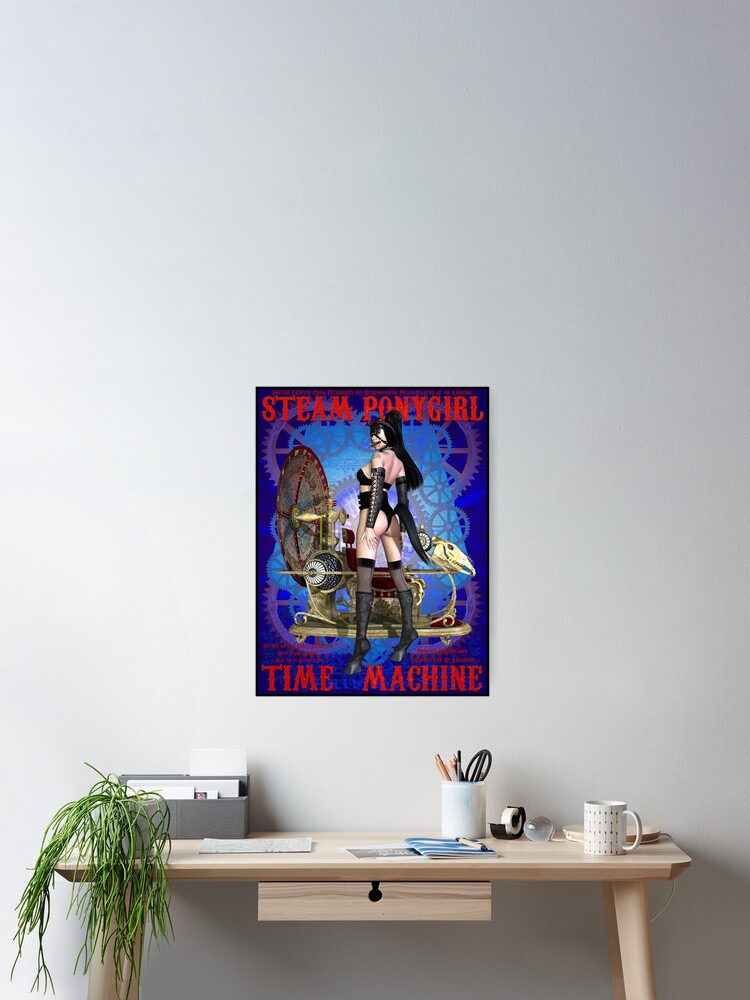The image depicts a small, simple home office setup against a white wall. A slim, natural wood-colored desk with a single drawer sits in the center. On the left side of the desk, a plant with cascading leaves reminiscent of a weeping willow adds a touch of greenery. Centrally placed is a white mug filled with pencils, pens, and scissors, while on the right side, another white coffee mug rests. An elbow-shaped white lamp stands on the desk, providing a modern touch. Above the desk, a poster prominently displays bold red lettering with the titles "Steam Pony Girl" at the top and "Time Machine" at the bottom. The poster features an illustration of a buttoned-up woman wearing steampunk attire, including a corset, bra, boots, and goggles, standing next to a steampunk contraption with visible gears and a seat. A box filled with papers can also be seen on the desk. The overall scene evokes a clean, organized, and slightly artistic workspace.